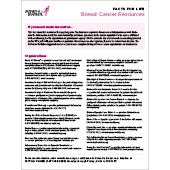This is a pixelated, low-resolution thumbnail image, likely designed for a newsletter associated with the Susan G. Komen Foundation, as indicated by the recognizable pink ribbon and the breast cancer awareness theme. The overall layout features a white background with black text and magenta-colored subtitles. The header, rendered in a lighter pink hue with a subtle gradient effect, spans the full width of the image. Below the header, the content is organized into two columns that presumably list various breast cancer resources. Unfortunately, due to the small size and poor quality of the image, the specific details in these columns remain illegible, except for the prominent text reading "Breast Cancer Resources." Toward the bottom, there's another expanse of text that likely includes additional contact information for the foundation's main offices, but the content is indiscernible.